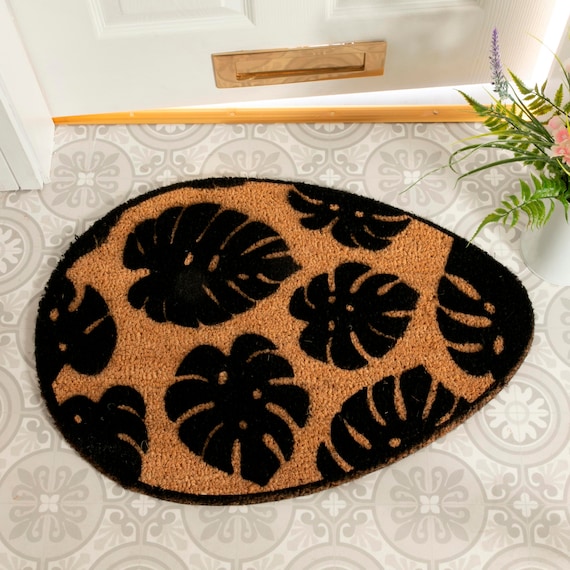The photograph captures a uniquely shaped doormat at the entrance of a home. The mat, resembling a sideways egg, features a black border with an orangish-brown background. Decorated with the silhouettes of large, elephant ear-like leaves in black, the doormat rests on an intricately designed tiled floor. The floor tiles showcase an elaborate pattern of gray and white floral motifs, including flowers and circular embellishments. In the top right corner of the image, a vibrant plant is positioned next to the mat, displaying lush green leaves alongside pink and purple blossoms. In the background, a white door, slightly ajar, reveals a golden mail slot that adds a touch of elegance to the scene.